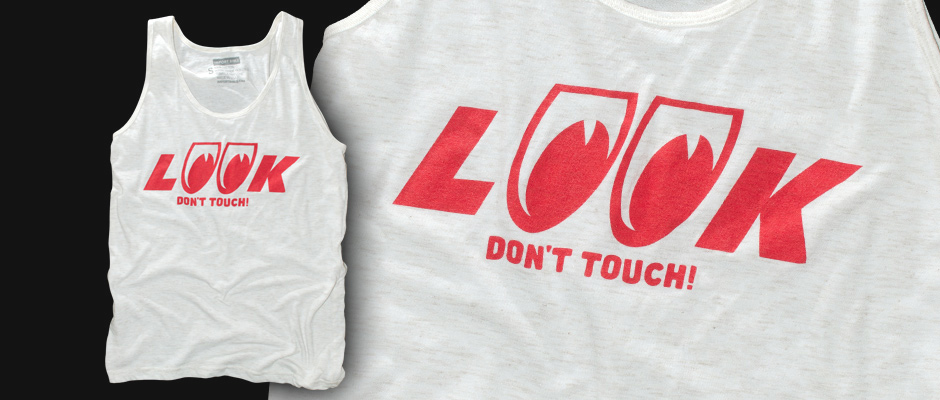The image showcases a white tank top against a solid black, rectangular background. On the left side of the image, there's a full view of the tank top, revealing its entirety from top to bottom, albeit extremely wrinkled with prominent lines and bumps. The tank top features a tag on its back. Centered on the front of the shirt is a striking logo that spells out "LOOK" with both O's designed as eyeballs, followed by "DON'T TOUCH!" in all capital letters and an exclamation point, all rendered in an orangish-red color. To the right, there's a close-up, zoomed-in view of the same logo, showing its intricate details clearly. This layout suggests a display style typical of online clothing stores, emphasizing both the full design and the detailed logo of the tank top.